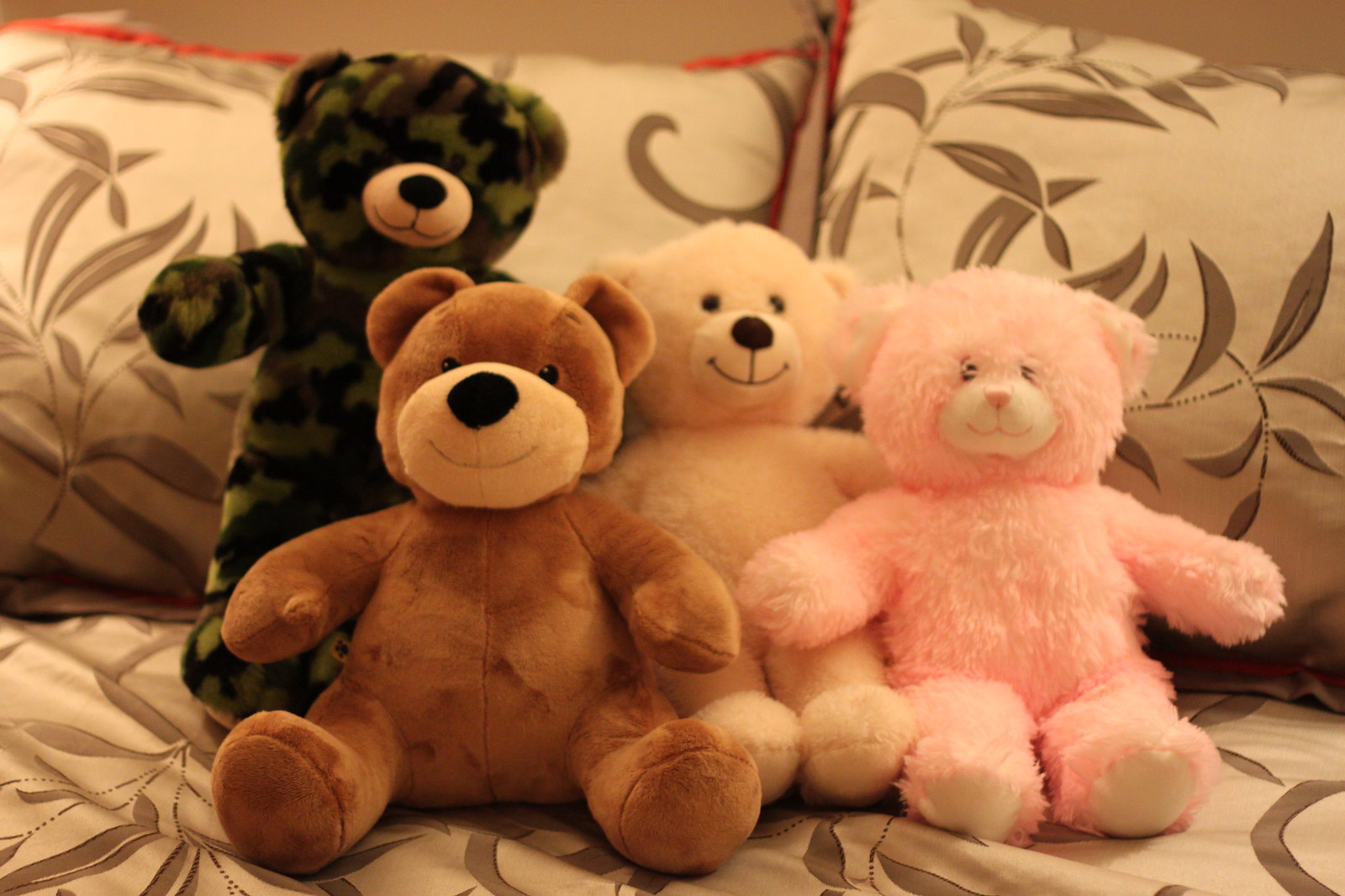This indoor photograph features a close-up of a bed adorned with coordinated pillow shams and a comforter, both showcasing a gray-green leaf pattern with red accents. Positioned in a neat row on the bed are four distinct teddy bears. The first bear stands out with its camouflage design in shades of olive, light, and dark green, complemented by a tan snout with a black nose and stitched mouth. The second bear is a rich chocolate brown with black eyes, a black nose, and a delicate black mouth on its tan face. The third bear is a soft peach color, boastin a tan face, black eyes, a black nose, and a matching stitched mouth. The final bear, strikingly almost hot pink, sports a pink nose and mouth, black eyes, and white pads on its feet. The bears' varied colors and designs create a charming and whimsical ensemble against the elegant floral backdrop of the bed linens.